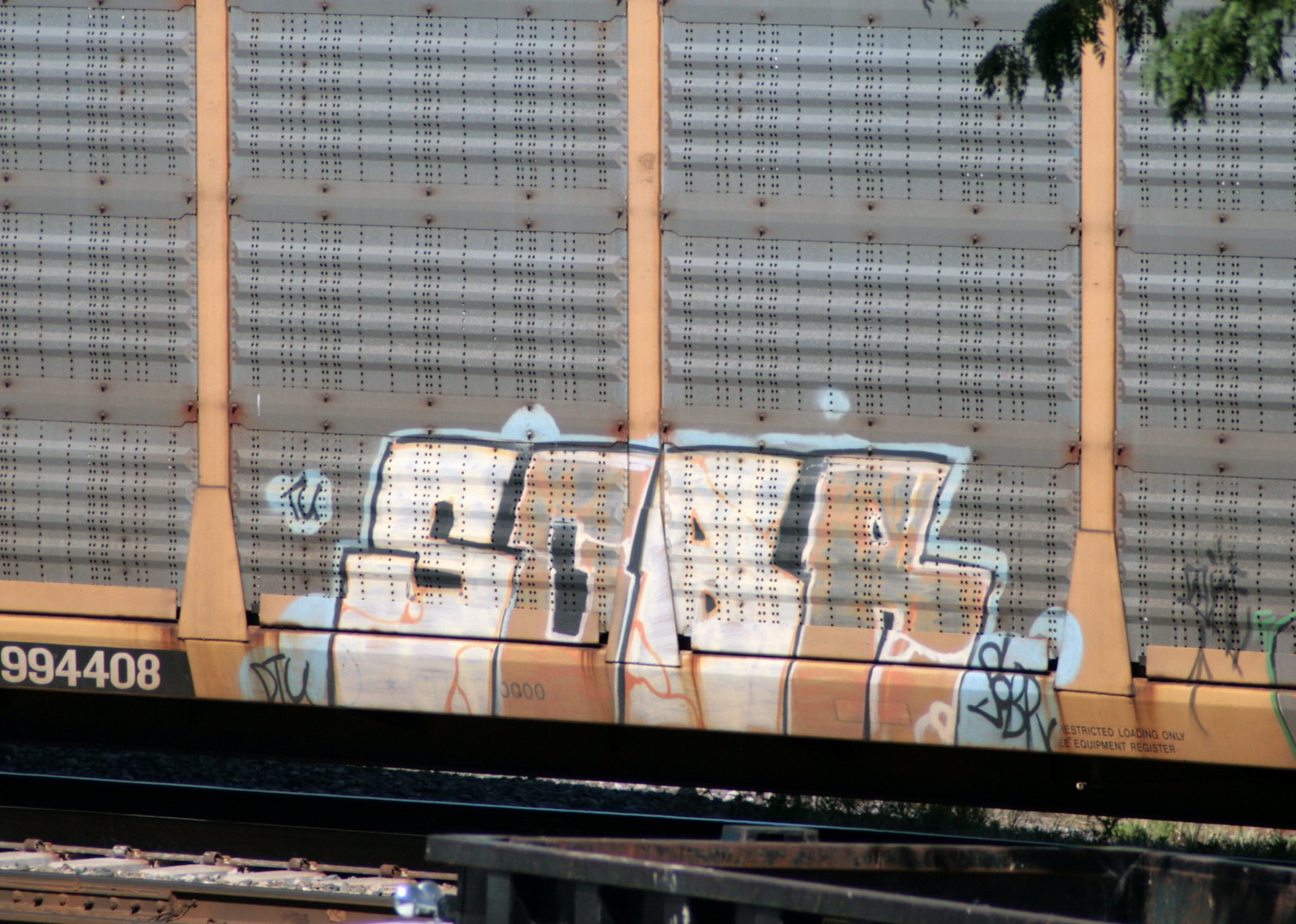The photo captures the side of a rail car featuring a detailed tableau of graffiti and industrial design elements. The rail car's metallic gray exterior is adorned with orange vertical beams, adding structural integrity and a touch of color. Dominating the lower half of the car, intricate graffiti spells out the word "SOAR" with bold, chunky letters: a white "S," a sand-colored "O," a white "A," and a white "R," each letter accentuated by a black outline and a unifying blue contour. Above the graffiti, the surface exhibits a paneled texture riddled with small holes, configured in a four-grid pattern. On the left side of the car, the number "994408" is prominently displayed, accompanied by the text "Restricted Loading Only, Equipment Register" near the bottom right. Surrounding the rail car, the setting includes visible sections of steel bars and rail tracks at the bottom, with a hint of greenery and small leaves peeking from the top right corner, adding a natural contrast to the industrial scene.